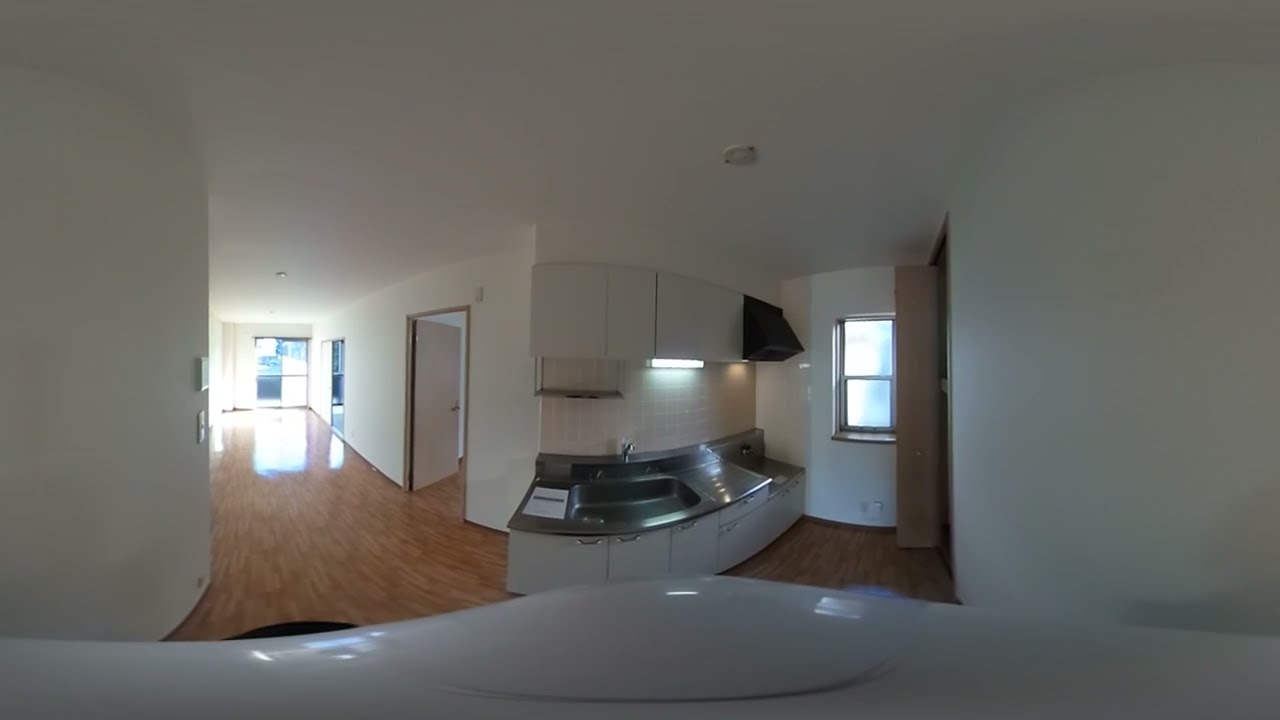The wide rectangular panorama photograph captures the interior of an empty apartment with striking clarity and brightness, accentuated by daylight streaming through the windows. The perspective, distorted by the panoramic lens, renders all straight lines as gently arcing curves, adding a unique sense of depth to the scene. The apartment’s walls are pristine white, contrasting with the light brown, glossy wooden floor that stretches across the space. 

On the left side, there is an orangey light brown door that appears curved due to the panorama effect. Adjacent to this door is a closet—its components also curved by the lens—with a similarly colored door. Beyond the closet, there are two sets of windows: one set with two rectangular panes stacked vertically and another with two rectangular panes placed side by side. From these windows, you can catch a glimpse of a tree outside, emphasizing it's daylight.

On the right side of the image, an open door leads into another room with the same type of shiny wooden flooring. At the back of this room, the entrance to a bathroom is visible, complete with a bath mat laid out on the wooden floor. The combination of white walls, brown hardwood floors, and the bright natural light creates an inviting and spacious atmosphere.